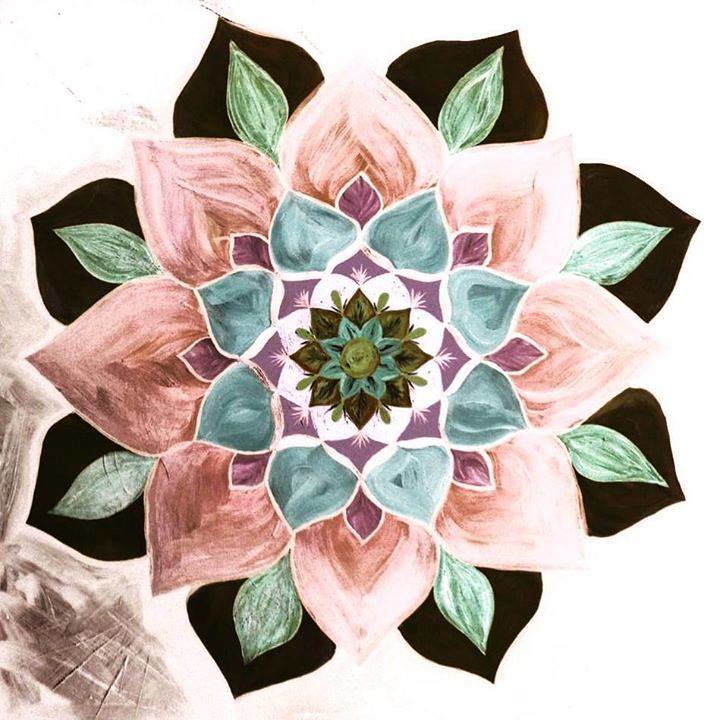This photograph showcases a meticulously drawn floral pattern, with intricate layers of petals nestling within one another. On the left side of the image, there are abstract floral scribbles rendered in pencil gray. From the outer edges moving inward, the petals transition through a variety of colors: starting with bold black petals, followed by vibrant green and white petals, and then a spectrum of mauve tones accompanied by various shades of pink. Continuing inward, the design features purple and gray-green petals, succeeded by brown and olive-green petals, and again interspersed with gray-green petals. The composition culminates in pristine white petals that encircle a deep forest green center. The image is of exceptionally high quality, capturing the crisp, clear details of the intricate design, and its large scale adds to its visual appeal.